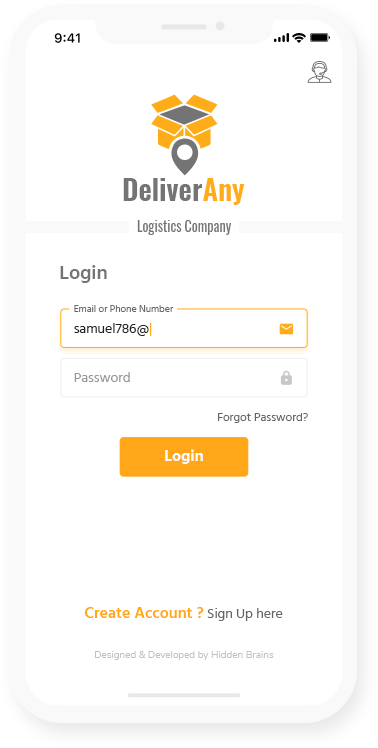In this image of a cell phone screen, the top-left corner displays the time "9:41." On the top-right, you can see four signal bars, volume bars, and a fully black battery icon. The top section has a shaded gray background, while the rest is white, providing a clear contrast for the time display. To the right, there's an icon of a person wearing a mask.

In the middle, there's a prominent orange box outlined in white, creating a 3D effect. The center of the box is dark gray, featuring a small search icon in dark gray, contrasting with a white center. Below this, in dark gray, it says "deliver," with the word "any" highlighted in orange, forming the phrase "Deliver any." Beneath it, "Logistics Company" is written in gray.

To the left, there is a "log in" option. The background remains all white, with an orange-outlined banner indicating the field for "email or phone number." The sample input shows "Samuel 786," though it's cut off. An orange envelope icon indicates an email address field. A gray banner below reads "password," accompanied by a small lock icon on the right. For users who may have forgotten their password, there's a "forgot password" link.

If the password is remembered, there's an orange banner at the bottom with "log in" written in white. Lastly, at the bottom of the screen, in orange, it says, "create account?" followed by "sign up here" in black. The fine print at the very bottom notes "designed and developed by Hidden Brains."